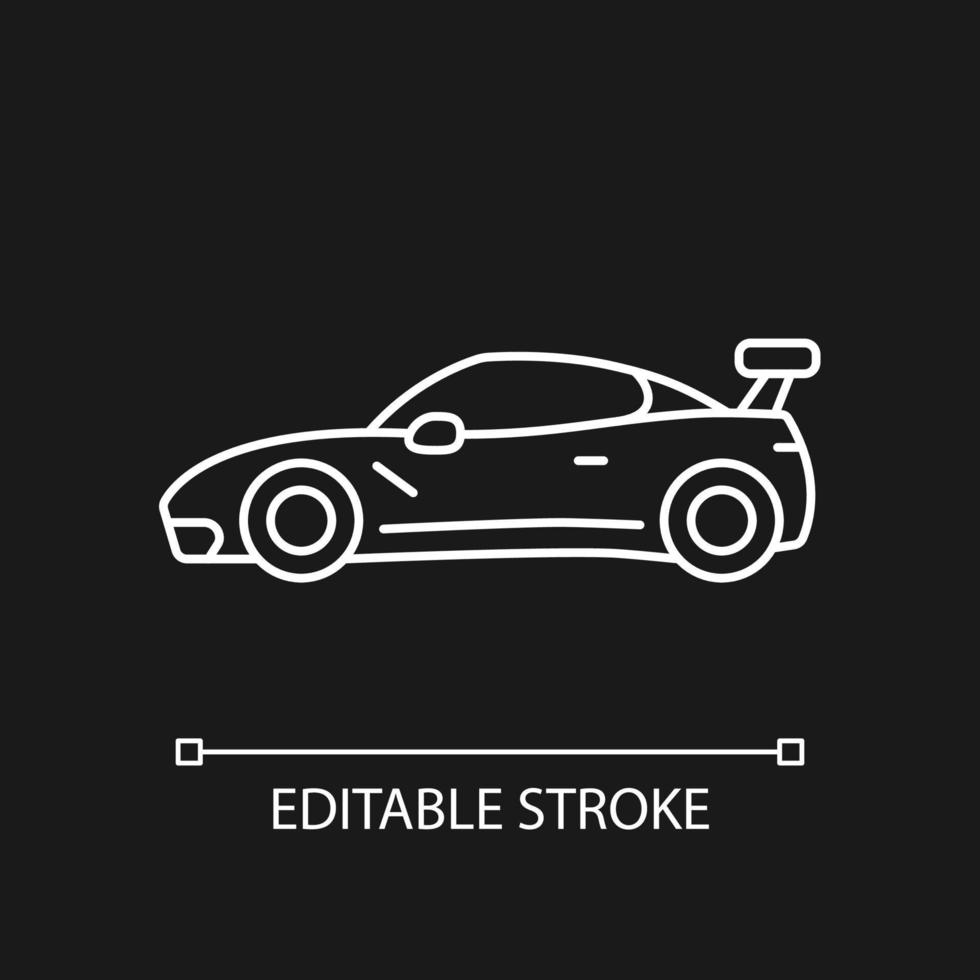The poster features a minimalist, computer-generated image of a sporty, four-seater car, rendered entirely in white against a black background. The car is presented as a simple line drawing, almost child-like in its simplicity but with clean, precise strokes that give it a chalk-like appearance. The car faces left, showcasing its side profile, including two even circles representing the wheels, smaller circles inside them indicating the hubs, and basic outlines of a rearview mirror and a window. Noteworthy details include a bumper and a streamlined spoiler above the trunk, adding a sporty touch. Beneath the car image is a horizontal line with tiny squares at each end. Below this line, the words "Editable Stroke” are displayed in white text, suggesting that the design is a prototype, possibly intended for further customization in advertisements.